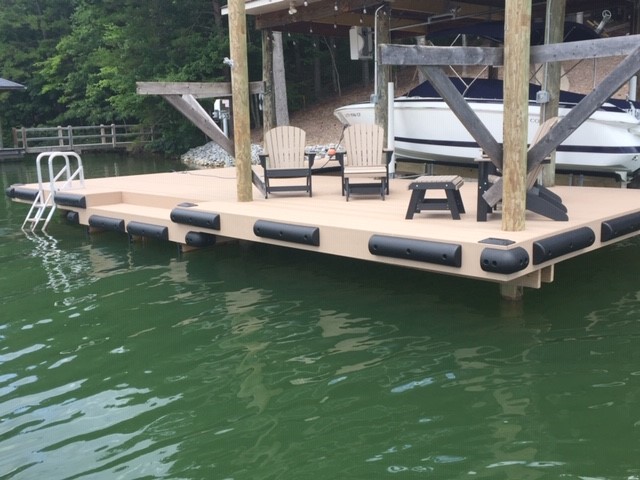The image captures a serene scene at a marina, featuring a floating wooden dock with various details that provide both functionality and aesthetic appeal. The dock itself is constructed from light brown wooden panels, complemented by beige columns and adorned with black and red markers around its perimeter, likely serving as bumpers to prevent boat collisions. The water surrounding the dock is a greenish-blue hue, with the dock stretching from the bottom left to the top left of the frame.

Prominent in the background, there's a white boat moored near the dock. Comfortable-looking beige chairs are arranged on the dock, though they are currently unoccupied. An inviting, almost tropical ambiance is further enhanced by a forested area with lush green trees visible in the top left corner of the image. Alongside the dock, there is a white swimming pool-style ladder that provides easy water access.

Anchoring the scene, large wooden posts protrude from the dock into the water, ensuring the dock remains stable. The shoreline is composed of a mix of gray rocks and vibrant green trees, illustrating a peaceful natural setting. Overall, the image paints a picturesque and inviting view of a tranquil marina, combining elements of relaxation and nature.